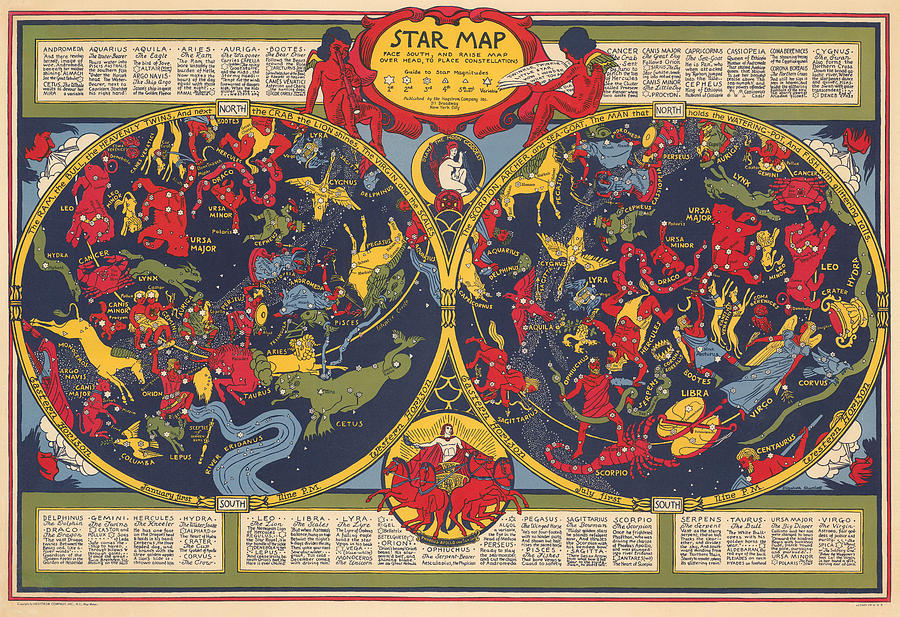This vibrant and vintage star map, designed with a 1970s or 1980s aesthetic, showcases a plethora of celestial bodies and astrological signs with intricate details. The map features a prominently oval-shaped header labeled "Star Map," adorned with two angels playing harps and spreading their wings. The dominant color palette includes olive green, periwinkle blue, red, and goldenrod yellow, complemented by black text. The map meticulously charts constellations such as the Big Dipper, Ursa Major, and Ursa Minor, alongside zodiac signs like Libra, Virgo, Scorpio, Sagittarius, Gemini, and Leo. Further enriching the display, it includes instructions on positioning the map during different times of the year, mentioning specific guidance for January and July, and highlights major stars and constellations including Andromeda, Aquarius, Aries, Cancer, Pegasus, and Taurus. The beige circles at the bottom detail various star constellations, emphasizing the north and south celestial hemispheres. This star map offers a nostalgic yet informative glimpse into the night sky, interweaving astronomy with astrology in a captivating visual presentation.